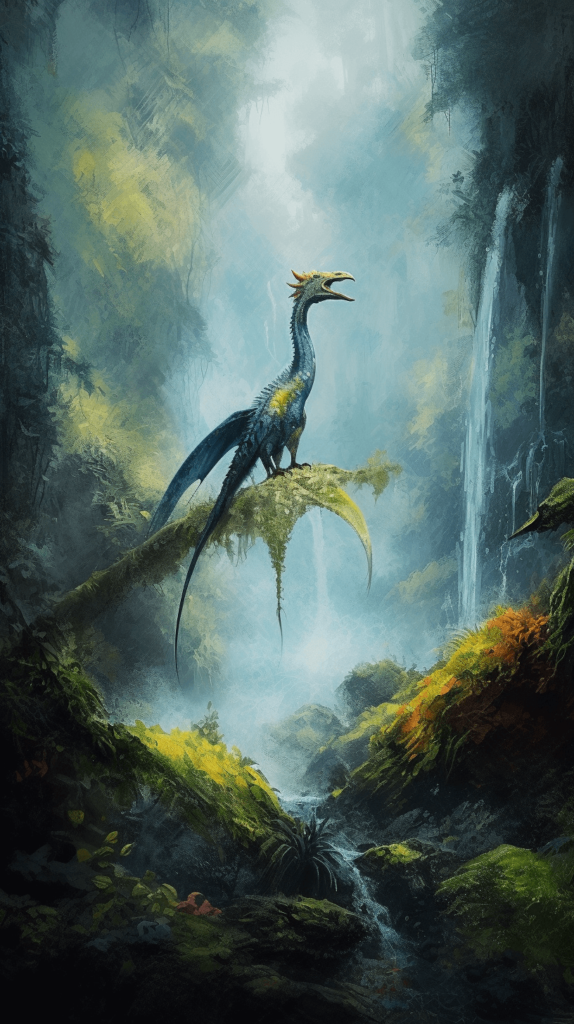The image is a detailed painting showcasing a prehistoric, possibly fantasy scene, dominated by a dinosaur-like bird perched on a moss-covered, fallen tree trunk that juts diagonally from the left side of the composition. The bird, dark blue with yellow accents and an open beak, gazes upward. It has at least one wing stretched backwards and a spiky ridge along its spine. The scene is lush and dense with vegetation, featuring vibrant green foliage, ferns, and moss, interspersed with touches of reddish-brown and orange plants. Below the branch, a small stream meanders through green and brown vegetation. The background is layered with a misty, wooded forest under a grayish, overcast sky, punctuated by multiple cascading waterfalls of whitish-blue water. The image exudes a primordial, almost mystical atmosphere with light filtering through the dense canopy, adding to its enchanting and ancient feel.